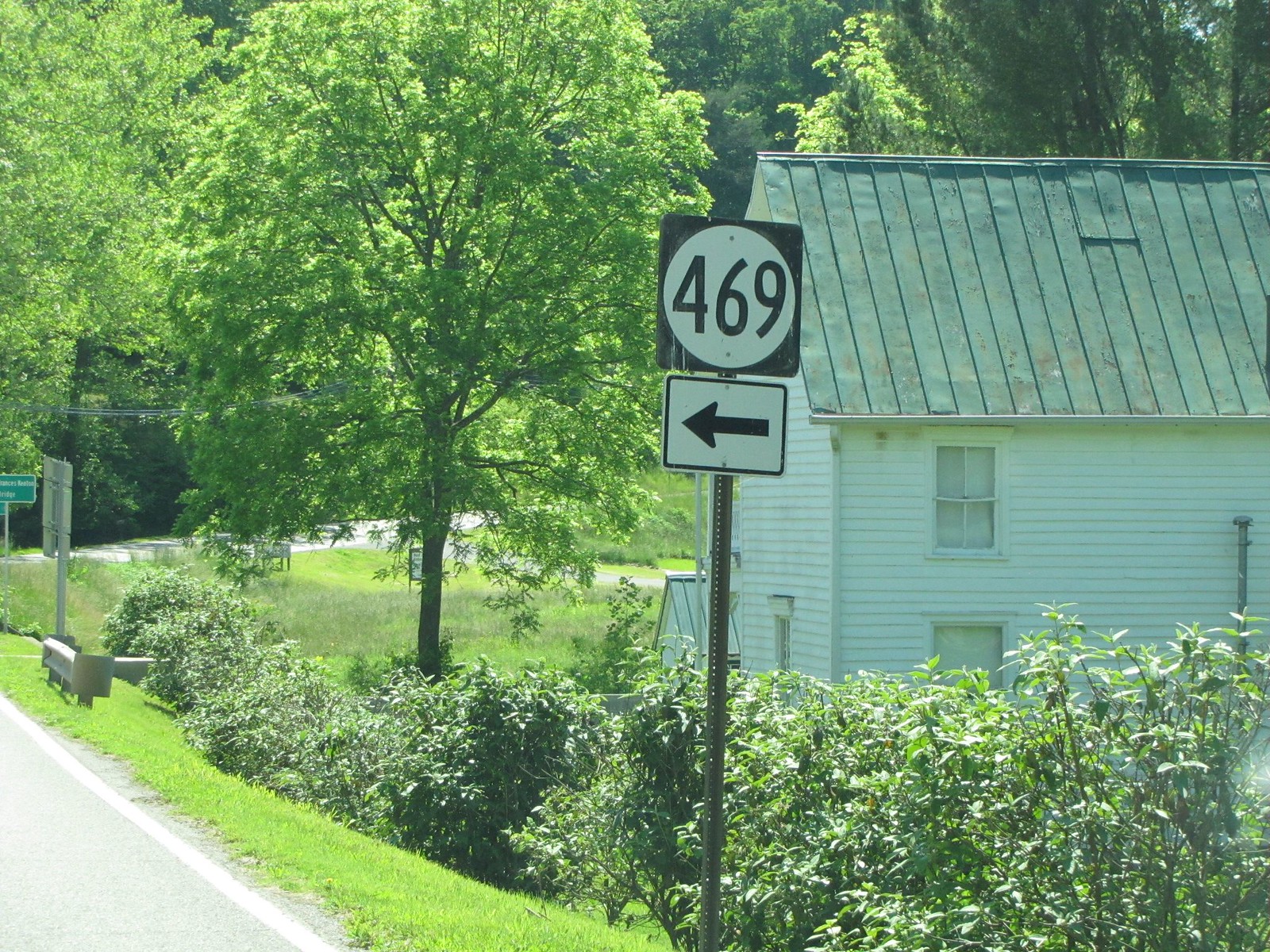This vibrant landscape photograph captures the beauty of a lush, green scene, characteristic of spring or summer. The background is densely packed with various shades of green trees, ranging from dark to light hues, creating a rich, natural tapestry. Prominent along the left-hand side of the image are thick bushes, which contribute to the picturesque setting.

In the bottom right corner, a stretch of road snakes into the frame, bordered by additional bushes that extend almost to the edge of the photo. Near this edge, a small guardrail subtly marks the boundary of the road.

Nestled amidst the hedges and in front of this verdant backdrop is a charming building with pristine white siding. The view shows the back of the building, displaying two windows—one on each floor. Its gray roof is adorned with long shingles that span from the top to the bottom, adding a distinctive texture to the building.

Adjacent to the road and slightly to the left of a large tree, a small door is just visible, adding to the quaint charm of the scene. Directly in front of the shrubs, a black pole stands holding a sign for Route 469. The white circular sign features black numbers and an arrow pointing to the left, directing travelers through this idyllic landscape.